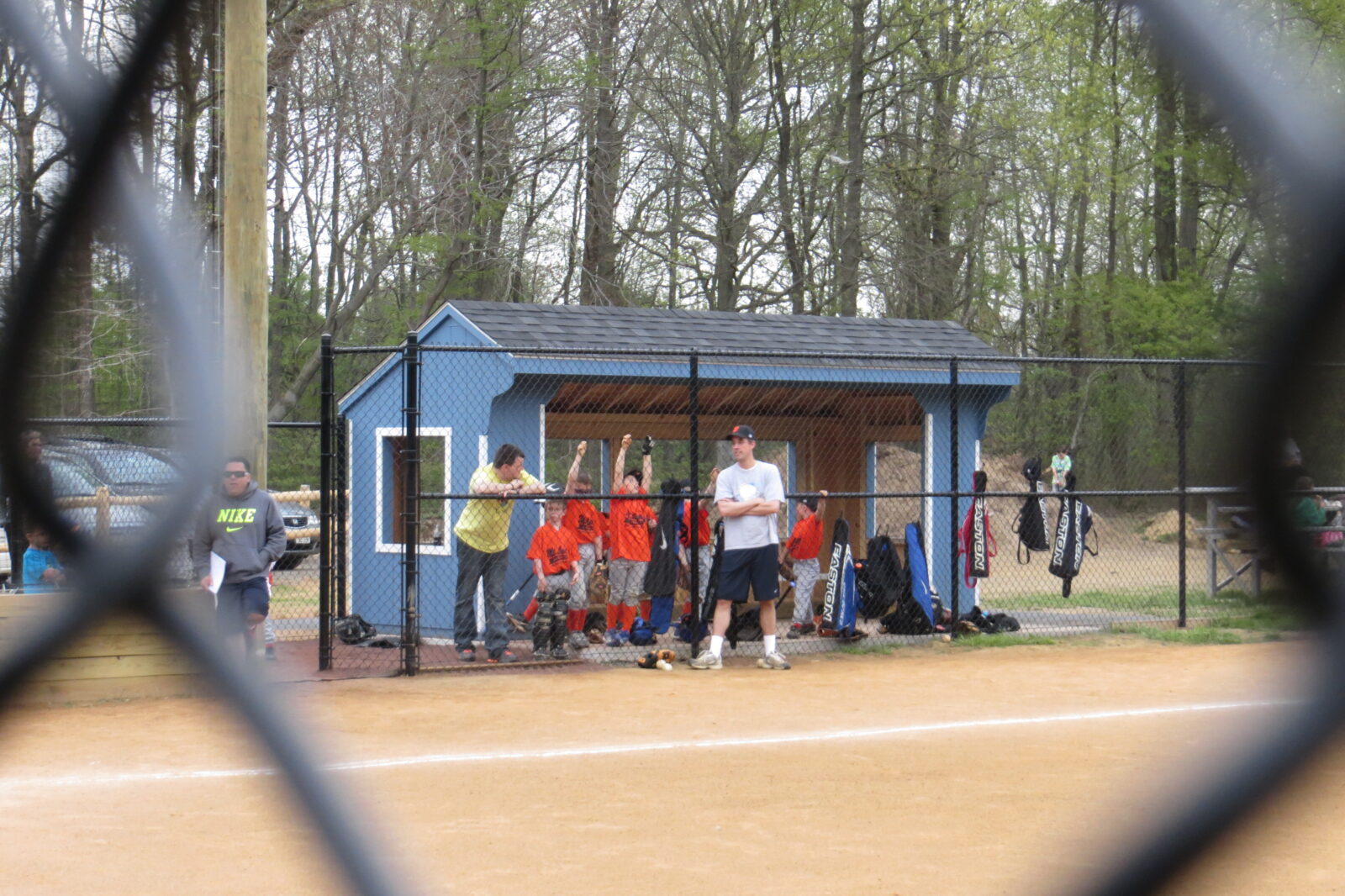This image captures a lively outdoor scene from the vantage point behind a chain-link fence, with the fence’s edges framing the picture on the left and right sides. In the center, a group of children, dressed in orange and light gray uniforms, are enthusiastically engaged in a softball or baseball game. Among them, some adults, presumably coaches, guide and supervise the young players. To the right of the field, behind another fence, a small blue wooden shed serves as the dugout. Several children can be seen inside the shed, preparing for their turn in the game. A notable adult figure, possibly the head coach, stands on the field with arms crossed. He is decked out in a black baseball cap, white t-shirt, black shorts, and white shoes, and his focused gaze is directed to the left, watching the game with intent. This vibrant scene exudes the energy and camaraderie of youth sports.